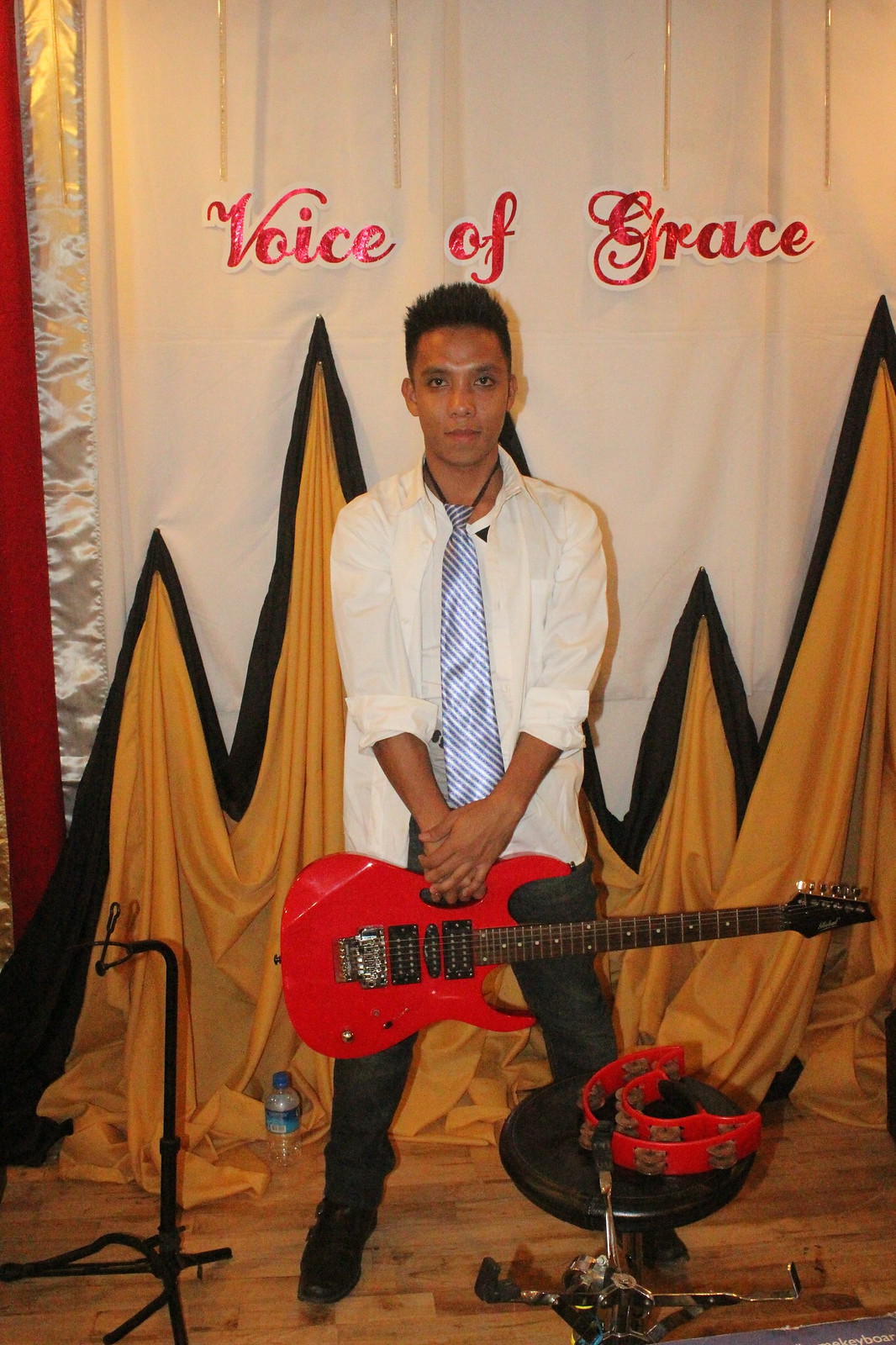The photograph captures a young male performer on stage, standing confidently with his feet shoulder-width apart. He has brown skin and dark black hair, shaved close at the sides and slightly spiky on top. His attire includes a crisp, white button-up shirt with sleeves rolled to the elbows and a shiny, blue and white striped metallic tie. He wears dark jeans and black shoes, and his untucked shirt reveals a T-shirt underneath. The man holds a striking red electric guitar, its vibrant color standing out against his white shirt.

In front of him, on the right side of the stage, there is a black stool with a red tambourine placed on top. Nearby, a metal drum stand with three prongs and another unidentified black stand can be seen. The stage floor is made of light brown wood planks.

Behind him, the backdrop consists of three layers of curtains: a white sheet with "Voice of Grace" embossed in pinkish-red script at the top, a lower black curtain, and an additional orange curtain with a black border. The setting is well-lit, emphasizing both the performer and the stage details, creating an engaging and professional atmosphere.